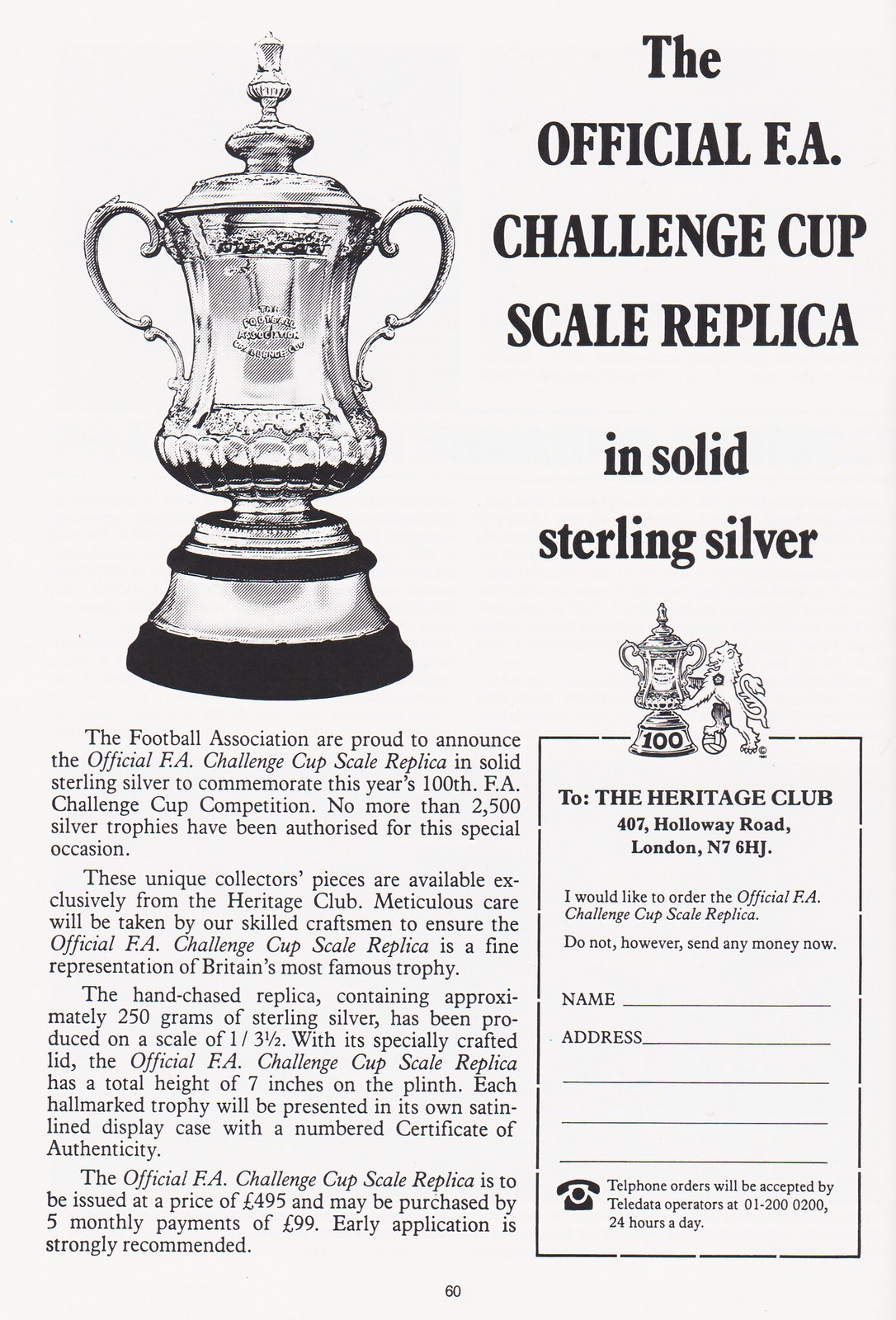The image is an advertisement and order form for the official FA Challenge Cup scale replica, crafted in solid sterling silver. The background is light grey, with multiple lines of black text. The top left corner features an image of the trophy, a grey chalice with a black base. The top right corner reads "The official FA Challenge Cup scale replica in solid sterling silver." Below this is text detailing the Football Association's announcement of the release of this scale replica to commemorate the 100th FA Challenge Cup competition. Limited to 2,500 authorized pieces, these unique collector's items are available exclusively from the Heritage Club. Skilled craftsmen will meticulously create each hand-chased replica, featuring approximately 250 grams of sterling silver and a scale of 1 to 3.5. The trophy, including a specially crafted lid, stands 7 inches tall on its plinth. Each piece will come with a satin-lined display case and a numbered certificate of authenticity. The special edition is priced at 495 euros, payable in five installments of 99 euros, with early application strongly recommended. An order form to the right instructs interested buyers to submit their name and address to the Heritage Club, located at 407 Holloway Road, London N76HJ, or place orders via Teledata operators available 24 hours a day at 01200 0200.